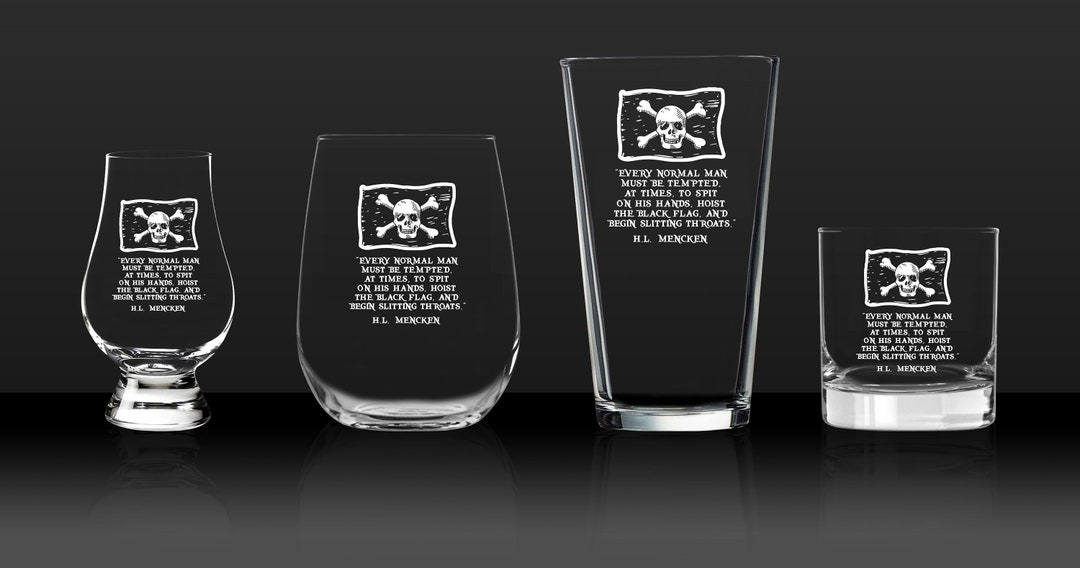This photograph showcases a collection of four distinct drinking glasses set against a stark black background and resting on a reflective black surface that mirrors their delicate forms. The array from left to right includes a chalice-style glass, a wine glass, a pint glass, and a whiskey glass, with the pint glass being the tallest and the whiskey glass the shortest. Each glass features a prominent skull and crossbones emblem, reminiscent of the pirate motif and akin to the iconic logos of NFL teams like the Oakland Raiders. Beneath the emblem on each glass is an inscribed quote by H.L. Mencken: "Every normal man must be tempted at times to spit on his hands, hoist the black flag, and begin slitting throats." The photograph emphasizes the clear, crisp detail of the glassware and the uniformity of the inscriptions, set against the dramatic blankness of the background, making the skull and crossbones emblem along with the bold quotation the focal points of the image.